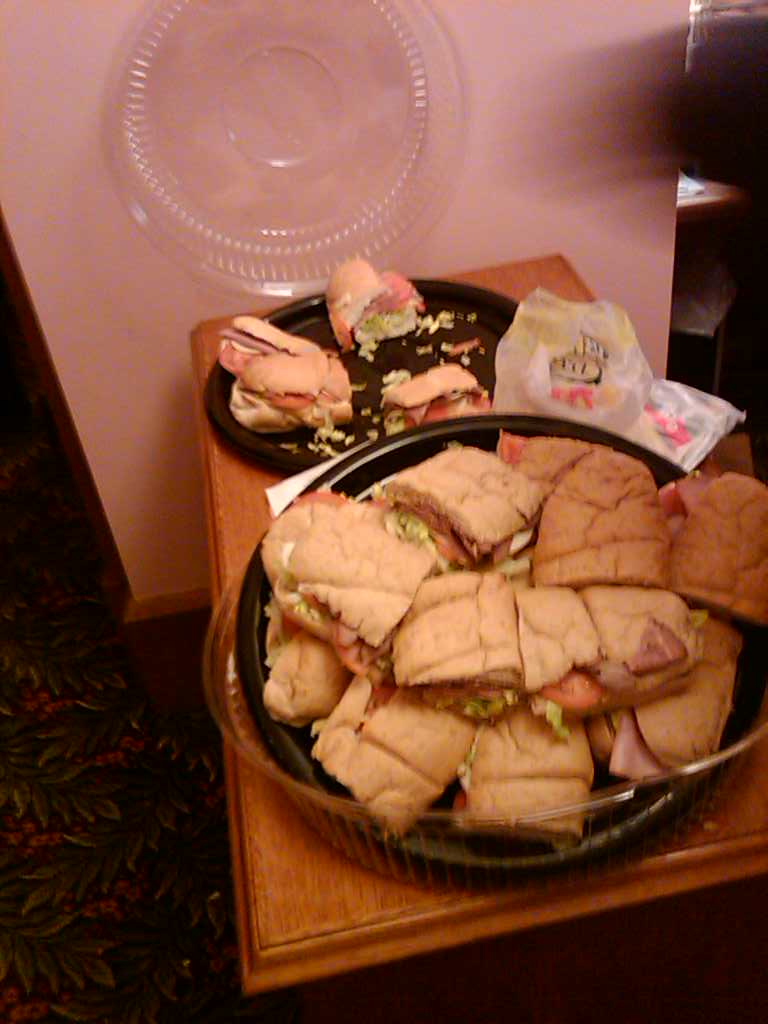This image is a color photograph capturing an overhead view of two takeout containers filled with bite-sized sandwiches. The sandwiches, which are unusual for their square shape, appear to be made from burger buns or a loaf with a textured top, featuring intersecting lines. Each sandwich is filled with lettuce, tomato, and possibly cold cuts. The containers are black with clear plastic lids; the larger container is placed upside-down while the smaller one is stacked perpendicular in the background. Both containers are set on what seems to be a wooden table, partially covered by a dark, floral-patterned rug. In the background, there is a partially visible white bag with colorful markings and a round plastic cover resting against a pinkish wall. A small light source, possibly from a window, illuminates the upper-right corner of the scene.